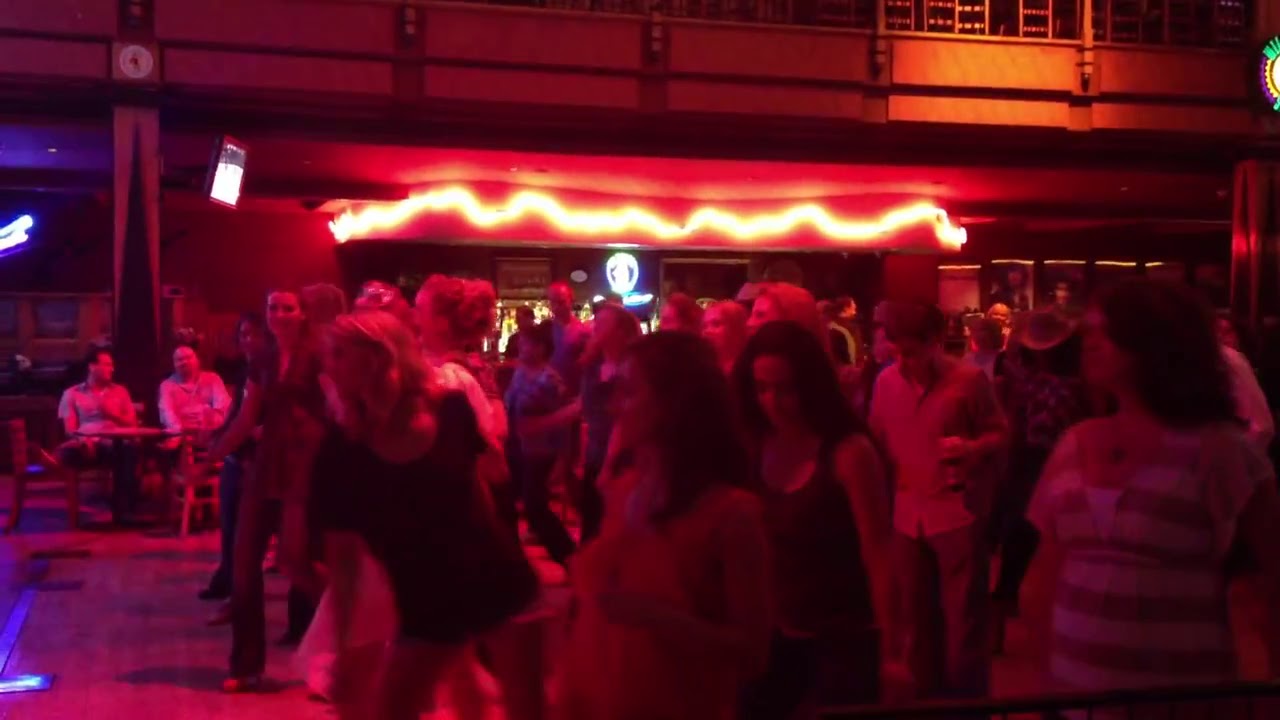The image captures a vibrant nightclub scene illuminated with an all-encompassing red glow, likely from a neon light strip that extends across the top of the bar. The club features a dance floor packed with a lively crowd, predominantly women but also a few men, appearing to engage in a form of line dance or simply reveling in the music. The motion and movement of these individuals render them slightly blurred, emphasizing their energy and the party atmosphere. A few people can be seen holding drinks, whether bottled or in cups, enhancing the festive vibe. In the background, there's a wooden balcony visible at the top of the photo, with the edges of some chairs just discernible. Near the back left side of the dance floor, a couple of tables with chairs are occupied by people engaged in conversation. The overall structure suggests a two-story venue, with the club likely occupying the ground floor, adding to the sense of depth and scale in the image.